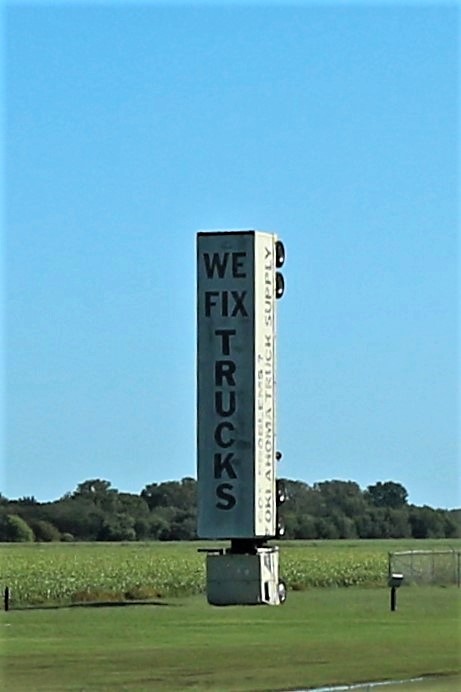Captured along a highway under a cloudless blue sky, this intriguing roadside sign features an 18-wheeler dramatically erected on its cab, with the trailer towering vertically behind it. The sign stands next to a burgeoning field of corn, not yet fully grown, and a dark-colored mailbox is noticeable to the right. In the distance, a line of trees frames the scenic agricultural backdrop. The trailer, adorned with bold black lettering, prominently displays the message "We Fix Trucks." Along its length, further information about the servicing company, which specializes in truck supplies, is detailed, making an unmistakable statement to passing motorists.